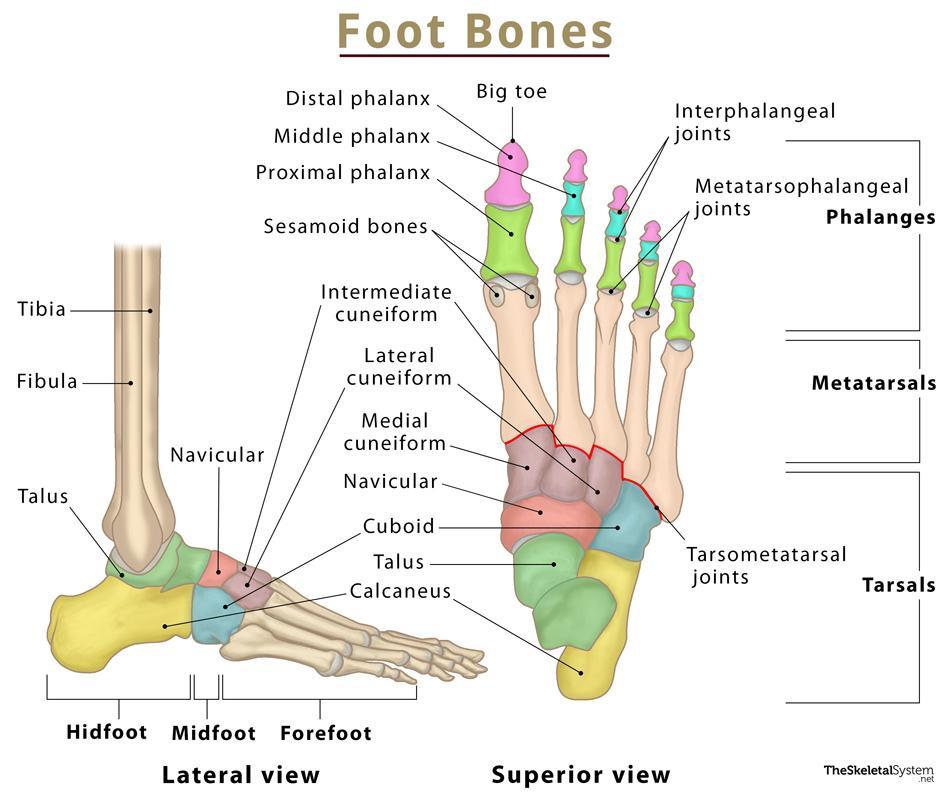This detailed diagram, likely seen in a doctor's office, prominently features the anatomy of a human foot, with the title "Foot Bones" written in gold, upper and lowercase letters at the top, underlined by a black line. The diagram showcases both a superior (top-down) view and a lateral (side) view of the foot. The bones are color-coded for clarity: the toes are highlighted in green with purple tips, while the main part of the foot includes various shaded areas in light purple, light red, light blue, light green, light yellow, tan, and beige. 

Each bone is meticulously labeled with words and arrows pointing to the corresponding structures. Central to the diagram, under the title, are the labels for the foot bones: distal phalanx, middle phalanx, proximal phalanx, sesamoid bones, intermediate cuneiform, lateral cuneiform, medial cuneiform, navicular, cuboid, talus, and calcaneus. Additionally, the interphalangeal and metatarsophalangeal joints, metatarsals in the middle section, and tarsals at the bottom are pointed out.

On the left side, another diagram provides a side view of the foot, extending to show the leg bones tibia and fibula. The terminology includes lateral view, superior view, midfoot, forefoot, and names of individual bones such as the tibia, fibula, and big toe. The diagram’s digital and informational style makes it an excellent educational tool, presenting an engaging and detailed visual study of the complex structure of foot bones.